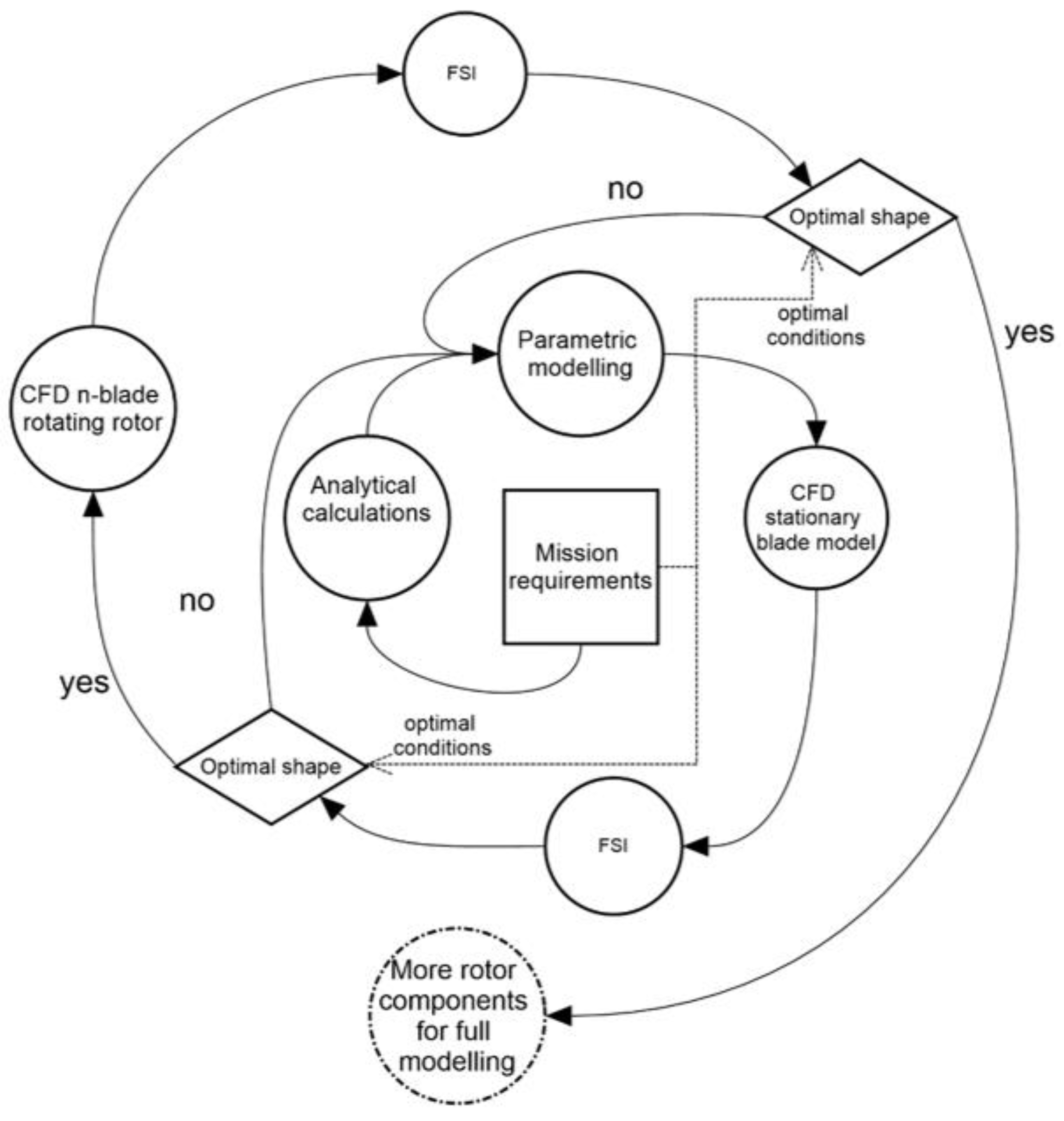This image depicts a detailed, computer-generated flowchart with a clean black-and-white design used for rotor design processes. The flowchart features various interconnected shapes, including circles, diamonds, and a central square, all with black outlines and filled with text in black. 

- **Shapes and Text:**
  - At the top, a circle labeled "FSI."
  - Midway, a square in the center labeled "mission requirements."
  - Diamond shapes labeled "optimal shape" located at the top right and bottom left.
  - Circles containing the text "CFD stationary blade model," "FSI," "CFD N-blade rotating rotor," "analytical calculations," and "parametric modeling."
  - A dotted circle at the bottom labeled "more rotor components for full modeling."

- **Connections and Flow:**
  - Arrows, some solid and some dotted, connect all the components. Diamond shapes have arrows indicating "yes" or "no" outcomes.
  - "Mission requirements" flow out to "analytical calculations" and an "optimal shape" diamond.
  - If "optimal shape" is not agreeable (No), the flow goes back to "parametric modeling."
  - If "optimal shape" is agreeable (Yes), it proceeds to "CFD N-blade rotating rotor," then to another "FSI," and circles back to an "optimal shape" check.
  - The final destination is "more rotor components for full modeling."

This flowchart meticulously outlines a rotor design process, beginning from mission requirements and concluding with full modeling of additional rotor components, emphasizing the checks for optimal shape at various stages.